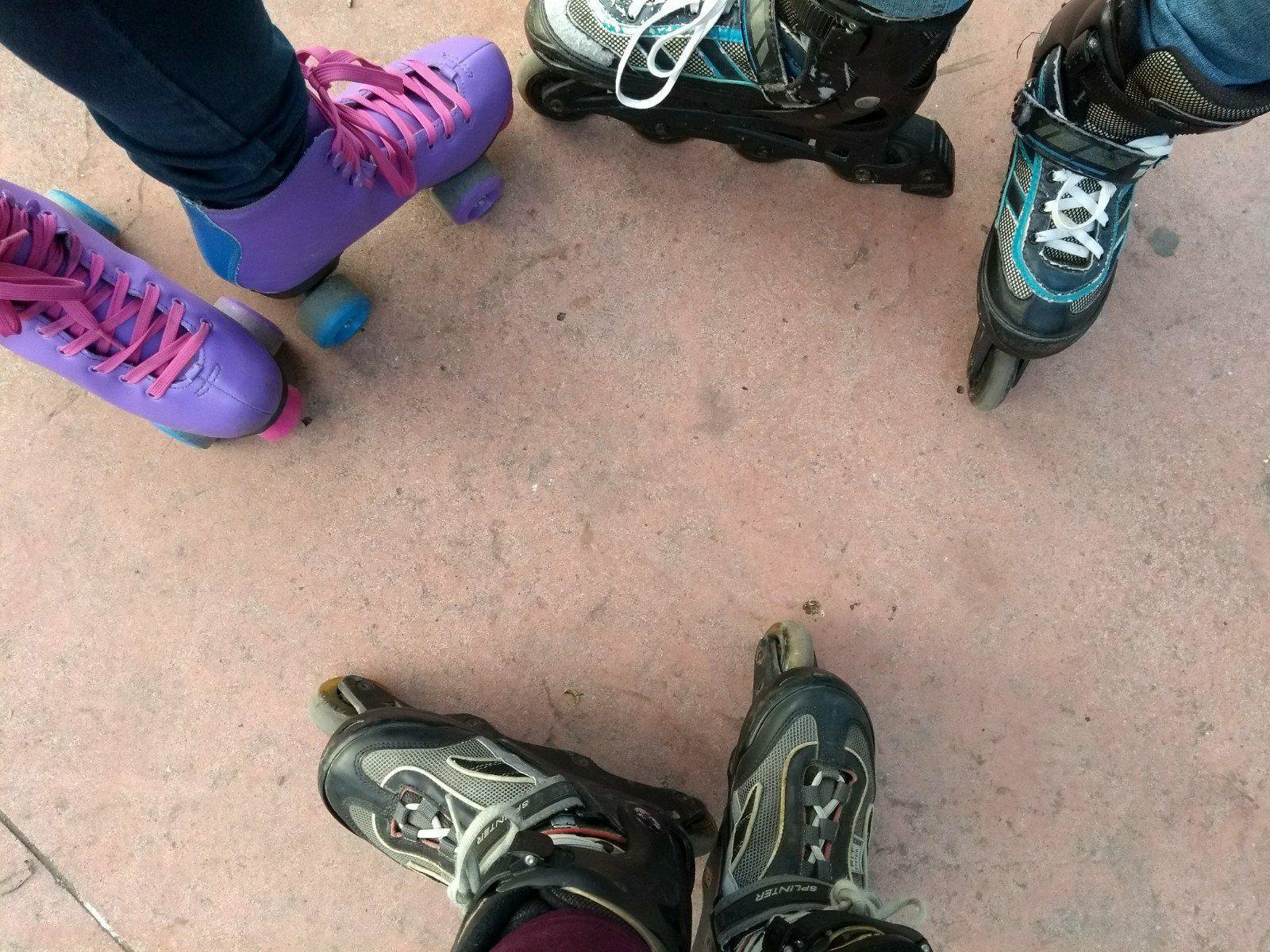In the image, the camera is looking straight down at the pinkish concrete floor, capturing the legs and roller skates of three people. The person in the upper left corner is wearing jeans and purple roller derby skates with pink laces, featuring an alternating blue and purple wheel pattern and pink stoppers. The person to the right is dressed in blue jeans and is sporting black inline skates with white laces, black heels, and light blue accents on the boot. The third individual, positioned towards the bottom, has on black, gray, and white inline skates with light brown wheels and a grayish velcro strap. They are standing on a pink cement surface that resembles a park or skating arena, illuminated by daylight.